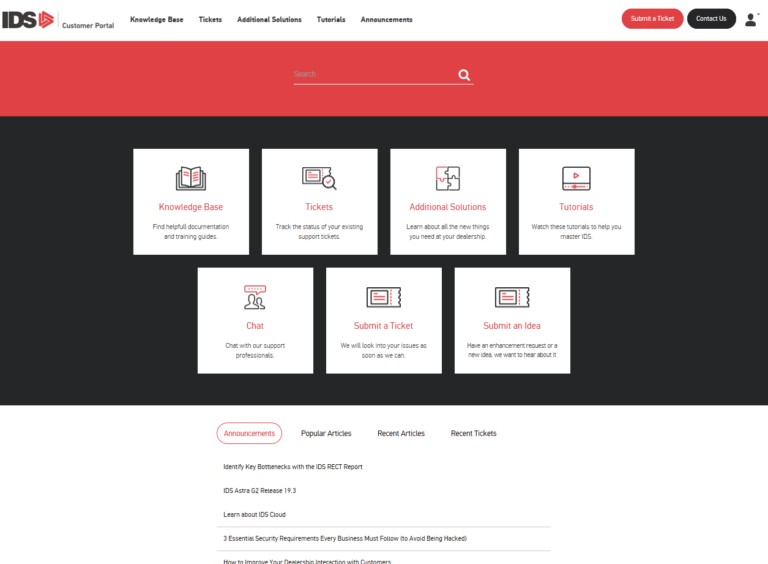The customer portal for IDS prominently displays its name in black alongside a distinctive reddish symbol. The portal features several sections, each easily accessible through its user-friendly interface. At the top, key headers such as Knowledge Base, Tickets, Additional Solutions, Tutorials, and Announcements provide a streamlined navigation experience.

Beneath these headers is a vibrant red search bar, complete with a magnifying glass icon, enabling users to quickly find pertinent information. Adjacent to this search bar, in the upper right-hand corner, are two prominent buttons: a red "Submit Ticket" button for reporting issues and a black "Contact Us" button for direct communication.

The main content on the page is set against a black background, which highlights seven white boxes, each representing a different functional area. These areas include:

1. **Knowledge Base**: An invaluable resource for finding helpful documentation and training guides, marked with a book icon.
2. **Tickets**: A section dedicated to tracking the status of existing support tickets, denoted by a ticket stub icon.
3. **Additional Solutions**: This area provides detailed information about new solutions relevant to dealerships, symbolized by interconnected puzzle pieces.
4. **Tutorials**: Featuring a video icon, this section offers numerous tutorials to help users master the IDS system.
5. **Chat**: Users can chat with support professionals for immediate assistance. This is indicated by a person’s icon.
6. **Submit an Idea**: This section encourages users to share enhancement requests or innovative ideas, also represented by a ticket stub icon.

Overall, the IDS customer portal is designed to be an intuitive and comprehensive resource for users, equipped with diverse tools to address all their support and information needs efficiently.